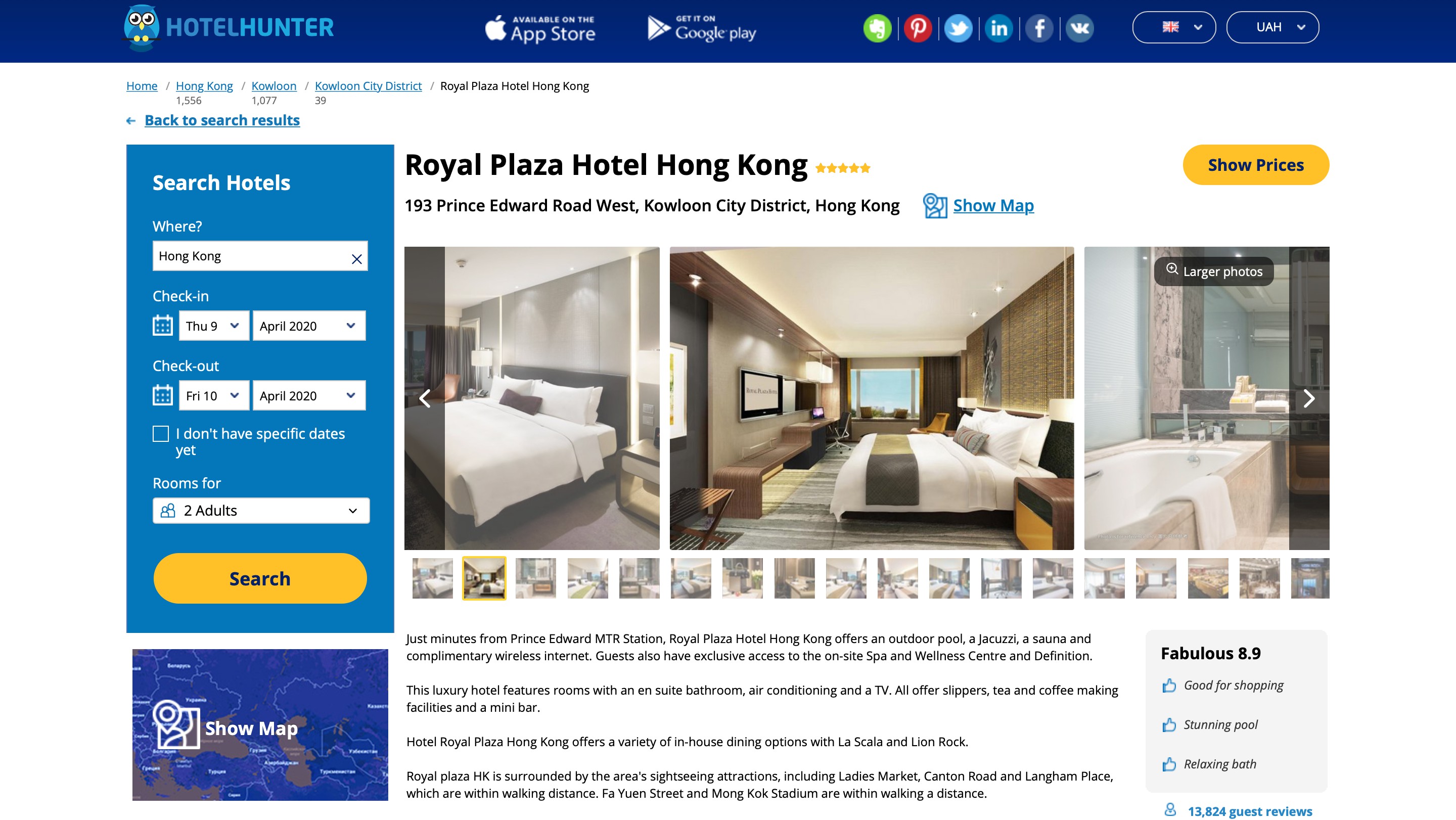The webpage for Motel Hunter displays a listing for the Royal Plaza Hotel Hong Kong, featuring three large images and several smaller images. On the left is an index with various tabs and options.

At the very top of the page is a navy blue banner showcasing an owl logo, accompanied by the text "Hotel Hunter" in two shades of blue. Icons for the Apple Store and Google Play are prominently displayed, as well as icons for Evernote, Pinterest, Twitter, LinkedIn, Facebook, and VK. Additionally, there is a British flag icon pointing downward indicating a language option, alongside another oblong icon marked "UAH" with a downward arrow, likely for currency selection.

To the left of the banner, breadcrumb navigation is visible: "Home" in blue, followed by forward slashes leading through "Hong Kong 1556," "Kowloon 1077," "Kowloon City District 39," and finally "Royal Plaza Hotel Hong Kong." Below this, a bold blue arrow directs users to "Back to Search Results."

Adjacent to this, a prominent blue button labeled "Search Hotels" is available. Underneath it, a search box labeled "Where" with a corresponding white input field invites users to specify their desired location.